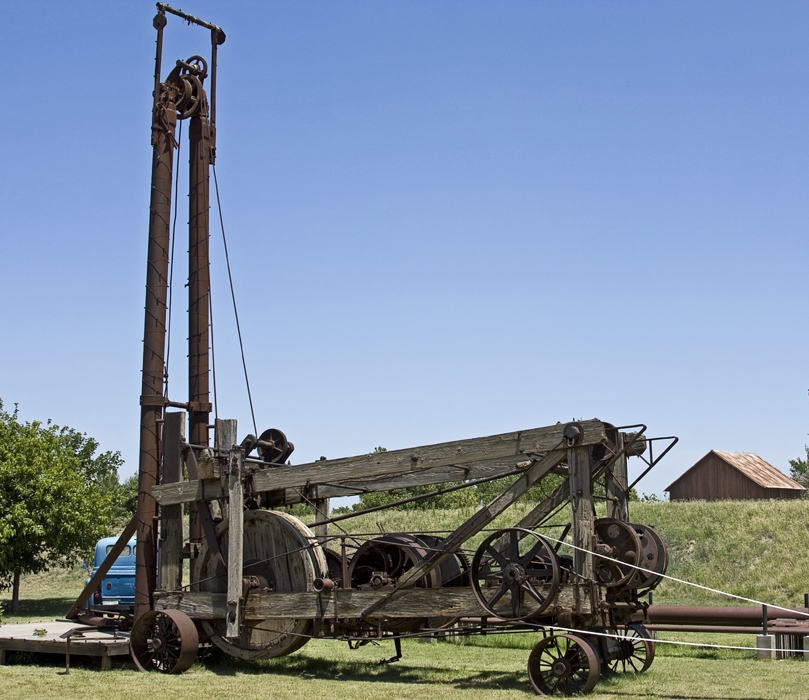The photograph captures a significant wooden contraption, likely an old piece of farm equipment, as its main focus. This tall structure, appearing to be around 20 feet on one side, features multiple metal gears, wheels, and belts integrated into its wooden rectangular frame. The contraption rests on four metal wheels and includes a complex pulley system with wires stretching from the top to the base. In the background, a weathered blue pickup truck is parked to the left, alongside a thin-trunked green tree. Behind the contraption lies a grassy field, a small wooden platform, and a gentle hill that ascends to a building resembling a house or barn. The setting is under a clear blue sky, suggesting a serene, rural environment.